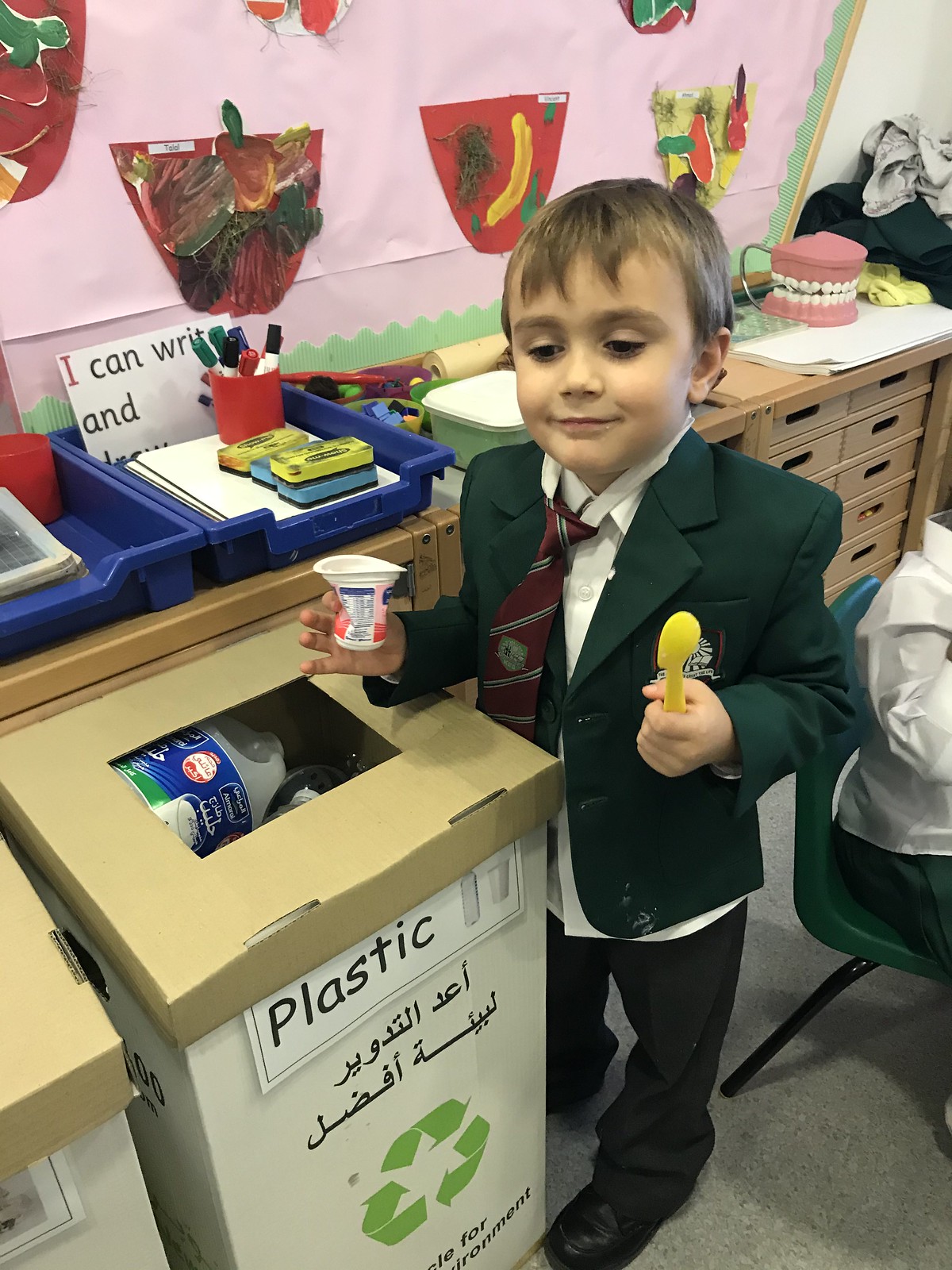In the photograph, a young Caucasian boy, approximately five to seven years old, stands poised to recycle. Dressed formally in an emerald green suit jacket over a white button-down shirt with a red patterned tie that is slightly askew, he holds an empty yogurt cup in his left hand and a bright yellow plastic spoon in his right. The boy, with light brown hair, is about to dispose of these items into a white plastic recycling container. The container, which has a brown cardboard top with a square cut-out, is clearly labeled "plastic" with black writing and the international recycling symbol. Other plastic items, including a bottle, are visible inside the bin. The setting appears to be a celebratory event or party, with pink walls and colorful decorations. Behind the boy, shelves hold various school supplies, a red cup holder with pens, and a decorative food item, possibly a cake, in pink and white. Despite the formal setting suggested by his attire, his focus on recycling underscores a moment of responsible action amidst the festivities.